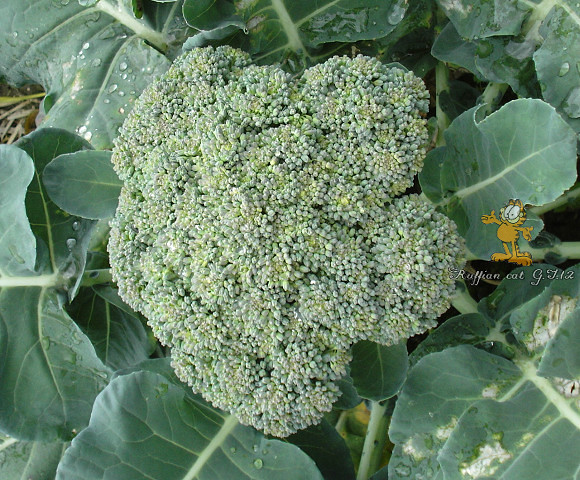An up-close, vibrant image primarily dominated by lush greens showcases a ripe head of broccoli at its center. The broccoli displays varying shades from a deep green to a slightly yellow-green on some crowns, with at least three or four distinct crowns featured. Surrounding the central broccoli head, radially arranged light green leaves glisten with water droplets, suggesting a recent rain or watering. The garden bed beneath is visible through the leaves, revealing a mix of grayish-brown soil and patches of hay or straw. In the bottom right corner, one leaf shows minor damage, yet the plant overall appears healthy and ready for harvest. Notably, to the right of the broccoli, a superimposed orange Garfield watermark with the text "ruffian.cat" adds a whimsical touch to the earthy scene.